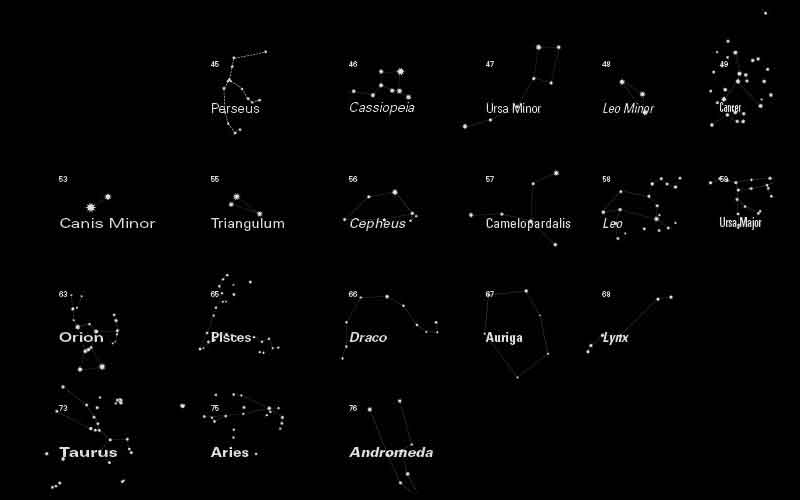The image features a black background displaying constellations organized in rows. The constellations are depicted as clusters of dots connected by lines, each labeled with its name in white font. There are four rows of constellations, with a few empty spaces. The first row includes Perseus, Cassiopeia, Ursa Minor, Leo Minor, and Cancer, with the first slot empty. The second row lists Canis Minor, Triangulum, Cepheus, Camelopardalis, Leo, and Ursa Major. The third row displays Orion, Pisces, Draco, Auriga, and Lynx, with one empty spot at the end. The fourth and final row features Taurus, Aries, and Andromeda, with the remaining slots empty. Each constellation is presented with its unique star pattern, ranging from a few dots to more intricate, connected designs. The top left corner and several spaces in the bottom row are notably empty.